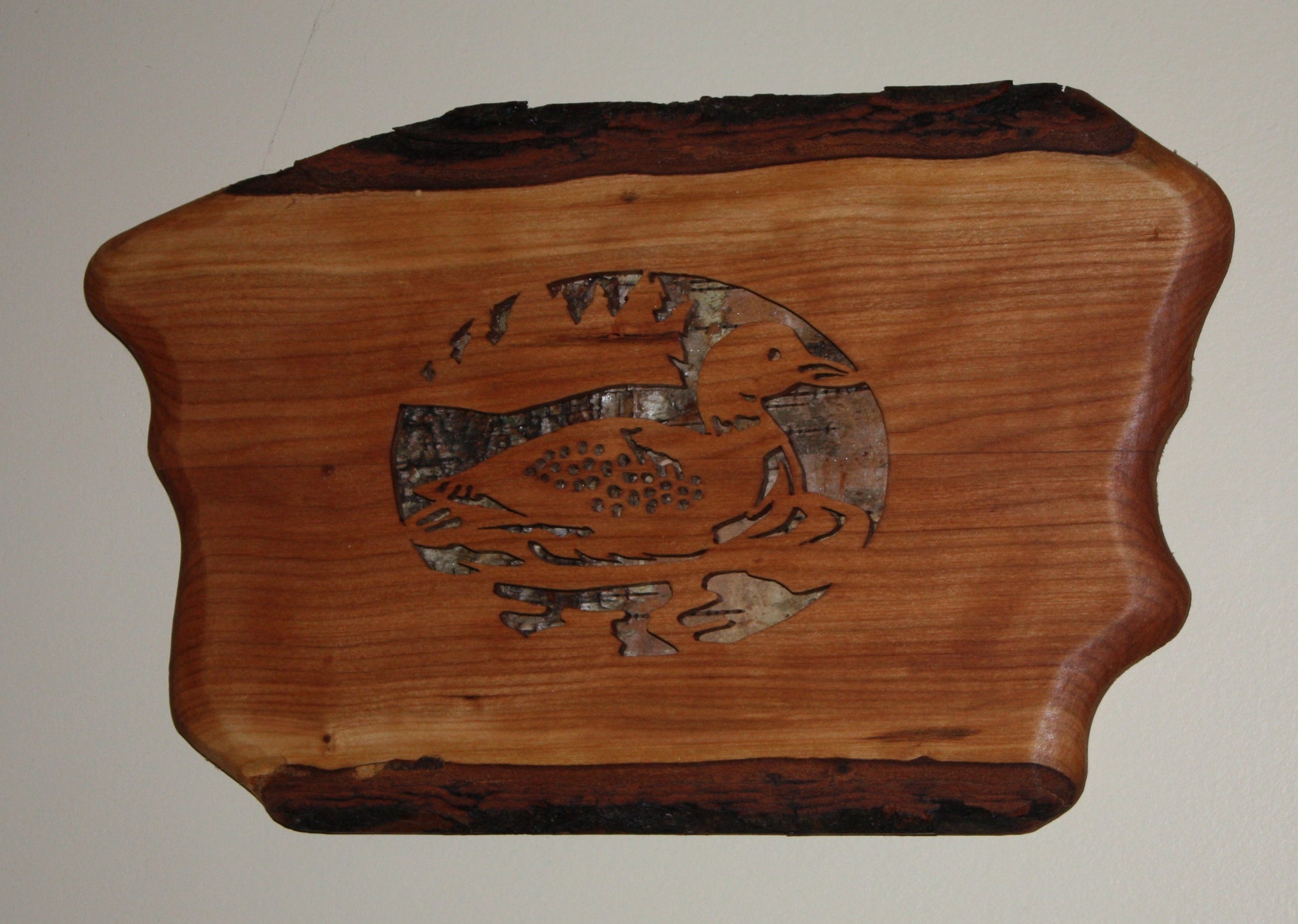This close-up indoor image captures a detailed view of a professionally worked wooden slab, shaped irregularly yet somewhat akin to an anchor, with an overall rectangular yet curved form. The slab exhibits a rich gradient of browns, showing a darker brown hue at both the top and bottom, transitioning to a medium brown that has been waxed to a smooth finish in the center. The slab, with several natural grooves and pointy corners on the edges, features an oval-shaped design in the middle, characterized by chipped-off sections with markings, including dots. This central design appears to be crafted from rotted wood, displaying a mix of black, white, and tan colors, possibly resembling pieced glass elements. The craftsmanship highlights both darker and lighter shades, presenting a cohesive yet intricate wooden artwork.